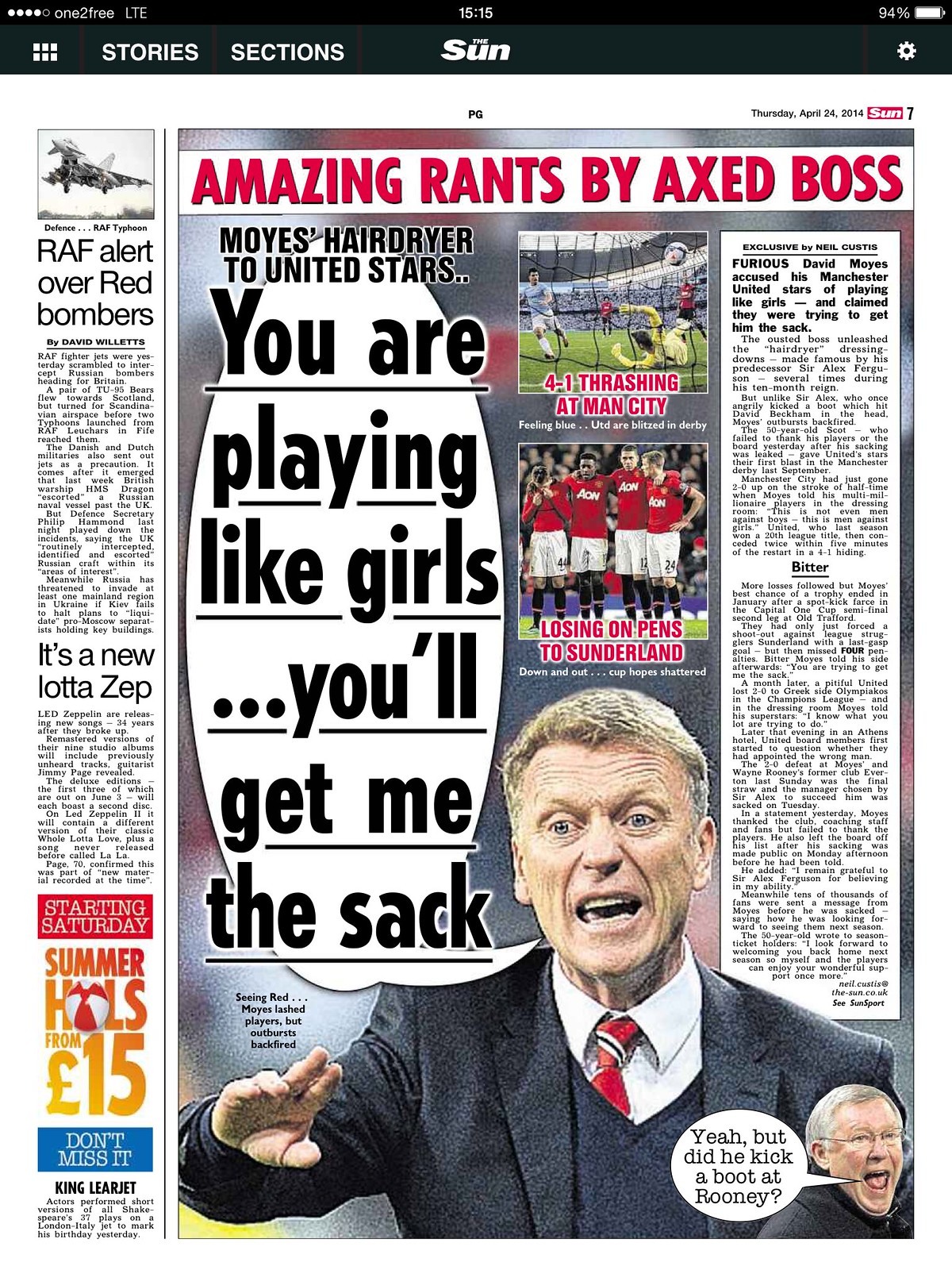The image is a screenshot of a vertically aligned sports-related article from The Sun, displayed on a mobile phone screen. The header of the article reads "Amazing Rants by Axed Boss" in bold, red capital letters. Below that, the subheading declares "Moyes Hairdryer to United Stars" followed by the striking quote, "You are playing like girls... you'll get me the sack," in large, bold, black letters. Dominating the visual is a photograph of a man, presumably Moyes, dressed in a suit with a vest over a white collared shirt, appearing to shout with his hand outstretched. 

Along the right side, there are two smaller images; above these photos, red text reads "4-1 thrashing at Man City," and below it, "Losing on pens to Sunderland." The bottom right corner features another small image of a man, with text that asks, "Yeah, but did he kick a boot at Rooney?" On the left side of the screen, a small subheading reads "RAF alert over red bombers" in black text, followed by an unreadable paragraph. At the very top of the mobile screen, a black bar displays the time "15:15," battery status, and connection indicators.